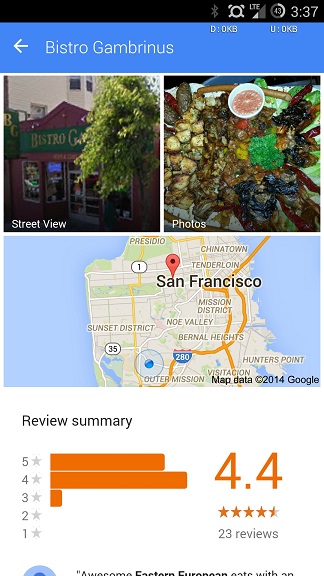A detailed screenshot of a cell phone is shown, focused on the Google Maps app displaying information about "Bistro Gambrinus" in San Francisco. The image, primarily consisting of the phone screen, is vertically oriented and cuts off about two-thirds down, seamlessly blending into a white background. At the very top is a black rectangular status bar indicating the time as 3:37 PM and connectivity details, including LTE and four signal symbols.

The screen reveals that the user has searched for "Bistro Gambrinus," spelled out as G-A-M-B-R-I-N-U-S. Below the search bar, there are two thumbnail images: on the left, a "Street View" showing the bistro facade with a tree in front, and on the right, under "Photos," a close-up of a table presumably laden with delicious shellfish. These thumbnails suggest further exploration, likely leading to more detailed images or views.

Below the visual previews, a map displays the location of Bistro Gambrinus in San Francisco, situated just to the west of the Tenderloin and north of the Mission District. Immediately following the map, the review summary is presented, showing an overall rating of 4.4 stars based on 23 reviews—signifying general approval with a slight skew towards 4-star ratings over 5. The screen captures the very top of a user review, with partially visible text hinting at praise for the restaurant's Eastern European offerings.

In essence, the screenshot offers a concise yet comprehensive snapshot of Bistro Gambrinus, aiding users in their quest for gastronomic delights in San Francisco.